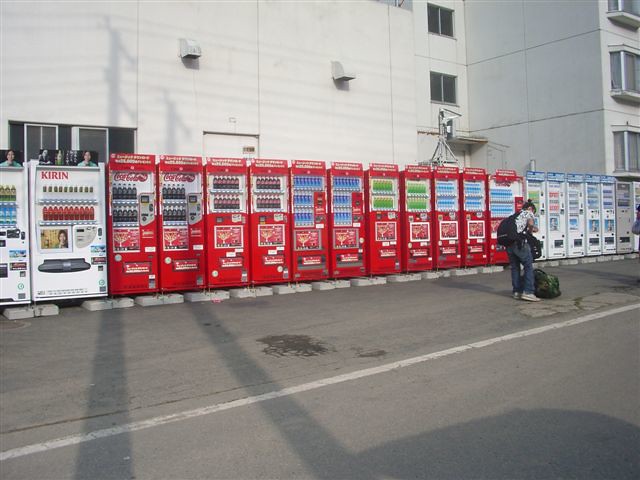This outdoor photograph showcases a white, multi-level building with several windows, situated alongside a two-lane asphalt road. In front of the building, forming a long, impressive row, are approximately 15 to 20 vending machines. On the far left, two white vending machines branded with "Kirin" in red letters offer blue, green, and red beverages. Following these are about nine distinctive red Coca-Cola vending machines, dispensing not only Coca-Cola but also bottles of green and blue liquids, likely various other drinks. The remaining machines on the right are white, slimmer than the ones on the left, and feature a blue header, although their specific contents are unclear. A person, standing off to the right of the image, faces the vending machines. Clad in blue jeans, white shoes, and a white shirt, they wear a backpack and have a bag at their feet, seemingly searching through another bag. The scene provides a peculiar yet detailed glimpse of an everyday setting, punctuated by an unusually large collection of vending machines.